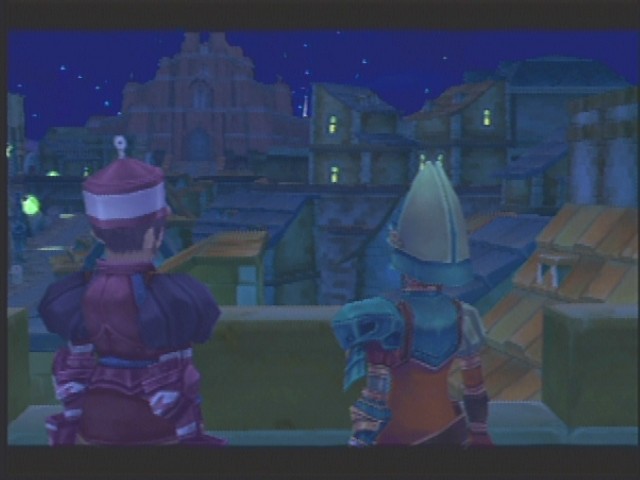This image captures a moment of gameplay featuring two characters standing atop a stone building, overlooking a sprawling city skyline. The first character has short brown hair and is dressed in a burgundy outfit with dark navy fluffy sleeves. They wear a distinctive burgundy hat adorned with a white stripe and a white ornament on top. The second character is equipped with a silver helmet and is clad in armor featuring shades of blue, brown, and silver. The building they stand on is made of silver and tan stone. The cityscape beyond them is a mix of red brick, tan, silver, green, and orange buildings. The backdrop is a night sky sprinkled with white stars, visible through various windows. Soft yellow light bathes the scene, adding a touch of warmth to the cool night atmosphere.